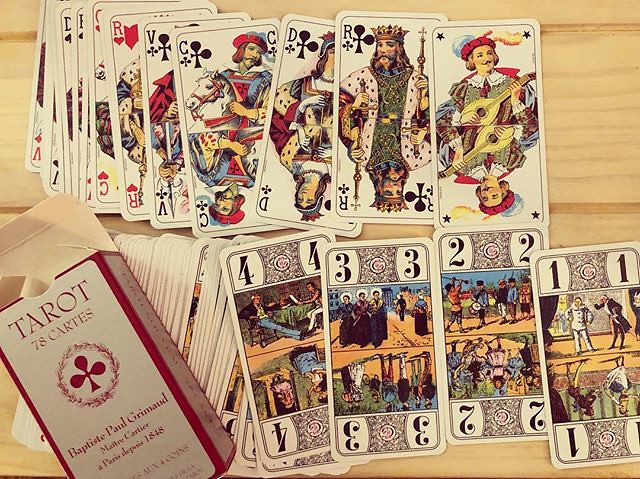A photograph captures a wooden table adorned with a scattered deck of cards. At the top of the image, a box labeled "Tarot Cards" is prominently displayed. The box also carries the text "Tarot 78" and "Baptiste Paul Grimaud," hinting that it might be in French. Contrary to the label, the visible cards resemble traditional playing cards rather than tarot cards. The upper section features face cards, including a Joker, King, Queen, and Jack, each exhibiting intricate, medieval-style sketches. The lower section displays numbered cards labeled one through four, continuing the medieval artistic theme. The overall scene is rich in detail, highlighting the craftsmanship of the cards.